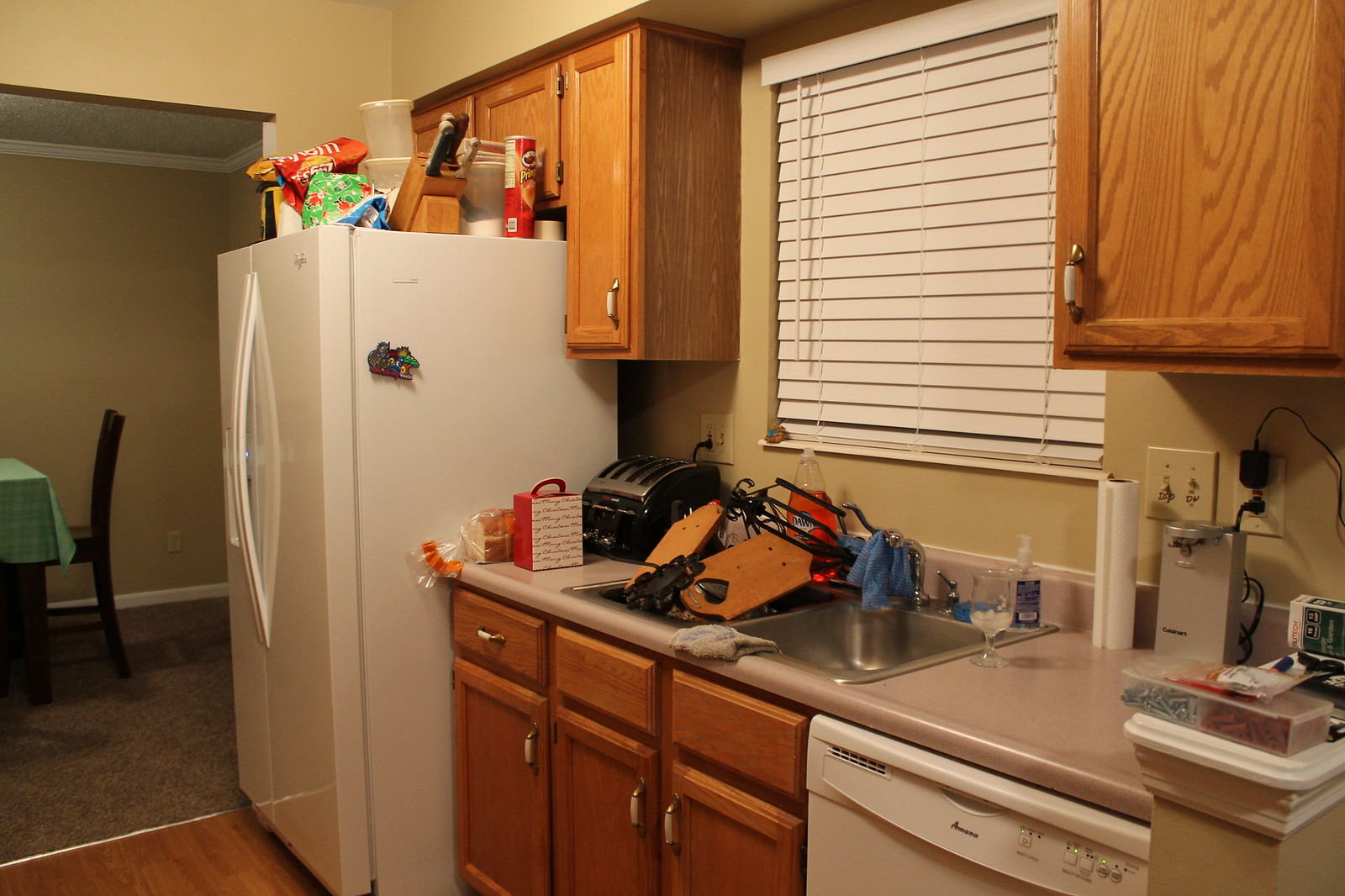This photograph captures a detailed view of a kitchen area focusing on the sink and its surroundings. The central feature is a gray or silver sink, filled with dishes on its left side. An orange-red bottle of Dawn dish soap sits prominently on the sink. Directly above the sink, a window with white blinds lets in natural light, flanked by light brown wooden cabinets with white handles. Below the sink are additional matching cabinets and a dishwasher to the right. To the left of the sink, there is a black toaster accompanied by a wrapped loaf of bread. Adjacent to this setup, a white refrigerator stands tall, adorned with a single magnet on its side. Atop the refrigerator, there are kitchen knives, a red bag of Lay's chips, and a red container of Pringles, adding splashes of color and a touch of casual clutter to the scene. The counter space to the right of the sink is occupied by various kitchen objects, contributing to the lived-in, functional atmosphere of the kitchen.